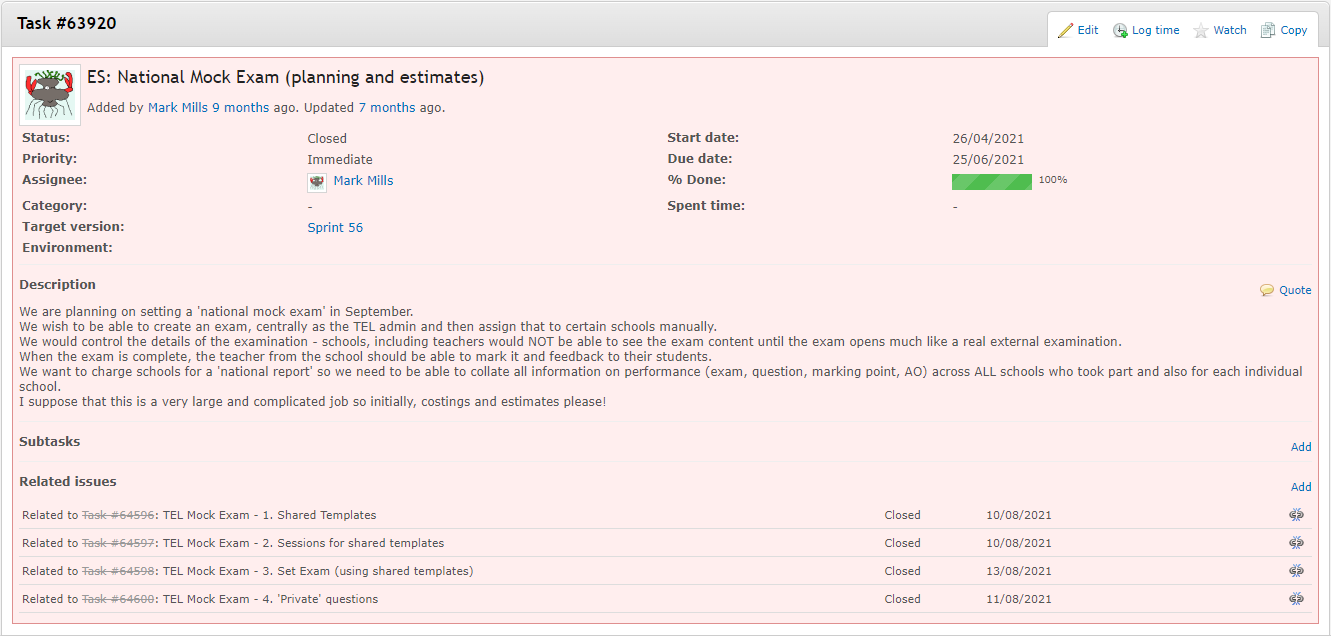Screenshot of a web page featuring a task management interface with a gray header. The header displays "Task #63920" prominently, alongside clickable options rendered in blue font including "Edit," "Log Time," "Watch," and "Copy." 

At the top of the task details section is the title "ES National Mock Exam Planning and Estimates," written in black font. Adjacent to it is a logo with red, gray, and blue elements on a white background. 

The task status is marked as "closed," and its priority is labeled "immediate." The task is assigned to "Mark Mills." Other details include: 
- Category: Blank
- Target version: Sprint 56
- Environment: Blank
- Start date: 04-26-2021
- Due date: 06-25-2021

The completion status shows 100%, highlighted by a green progress bar. 

The task description reads, "We are planning on sitting a national mock exam in September." Additionally, there is a section indicating related issues, listing four different mock exams, all of which have been closed.